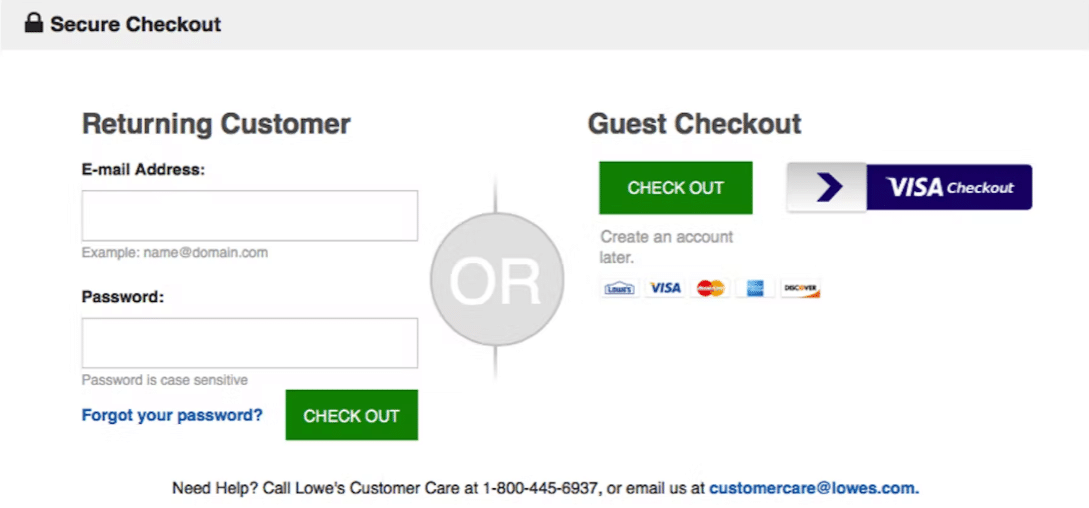The image features a secure banking interface for an online checkout process. At the top of the image, there's a gray, thin banner stretching from left to right with bold, black text that reads "Secure Checkout" beside a lock icon, signifying security. Directly below the banner, prominently displayed in larger black font, is the heading "Returning Customer." Following this heading, there is an email address input field. Directly underneath, there's a password input field with a note indicating that the password is case-sensitive. Below the password field, there's a link stating "Forgot Your Password?" with an adjacent "Checkout" button. Centrally positioned on the screen is a separator featuring the word "OR" inside a circle, flanked by horizontal lines above and below, indicating an alternative option. Below this separator is the "Guest Checkout" option, providing a clear and organized interface for different types of users.